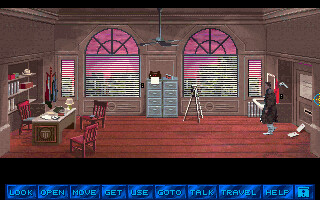The image appears to be a screenshot of an old 1980s-style video game, showcasing a detailed scene that might depict a library or a detective's office. The room features classic wooden paneling and a hardwood floor, adding to the retro aesthetic. A character, identified as a man wearing a brown trench coat and white pants, is seen entering the room from the left side. He appears to be walking purposefully across the room towards a desk on the right.

The space is furnished with multiple items: there are two wooden chairs with red cushions facing the desk, which also holds a lamp, a phone, and possibly a book. Numerous details, including two gray filing cabinets in the center, a tripod, and a bookshelf behind the desk, contribute to the rich setting. Dominating the back wall are two large arched windows with pink-tinted glass and blinds, enhancing the vintage feel. In the middle of the ceiling hangs a fan, further emphasizing the retro ambiance.

Furthermore, the bottom of the screen displays a blue banner featuring interactive buttons labeled "look," "open," "move," "get," "use," "go to," "talk," "travel," and "help," indicative of a point-and-click adventure interface. A small floppy disk icon is also present in the lower right corner, adding to the nostalgic impression of the scene.